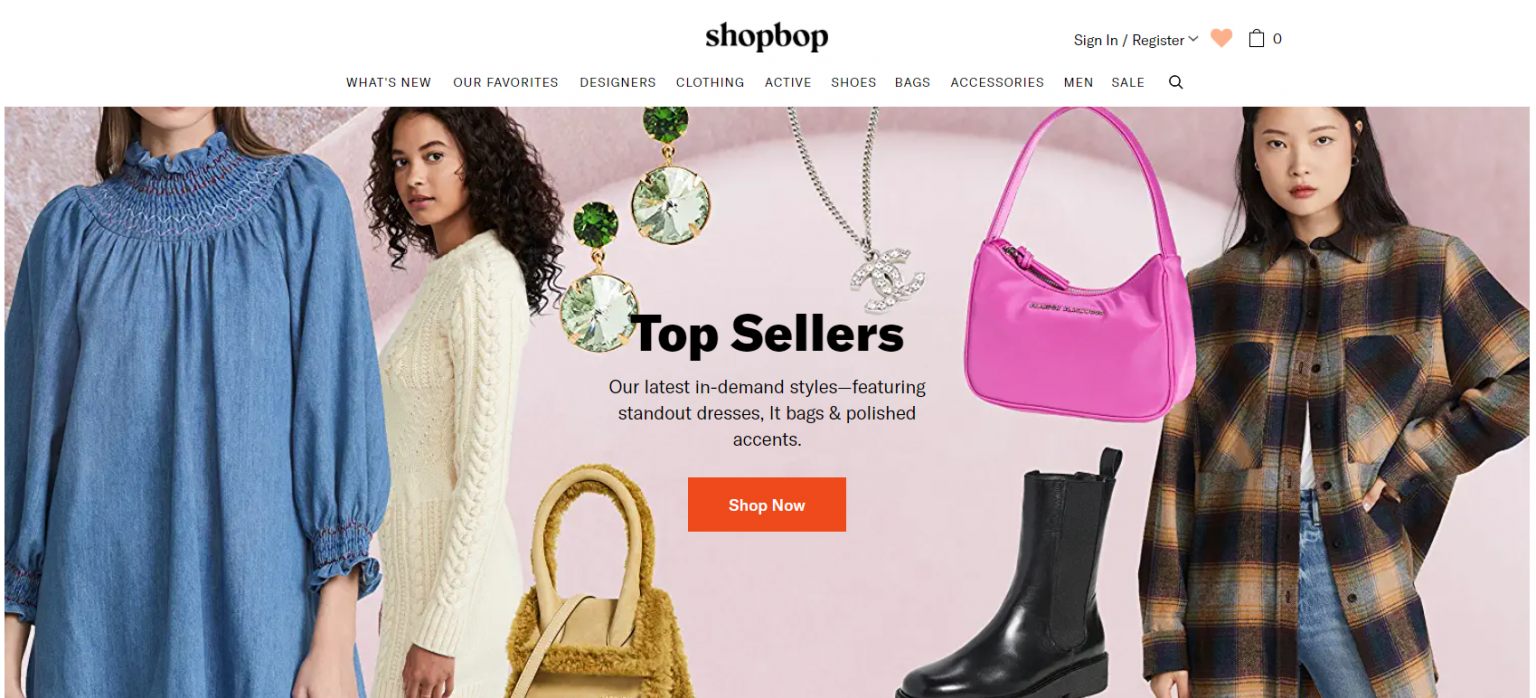The screenshot depicts the homepage of an e-commerce website named Shopbop, captured in a rectangular shape with the longer sides at the top and bottom. At the very top, a white banner stretches across the width. Centrally placed in this banner, the website’s name "shopbop" is displayed in all-lowercase black text. 

To the right of the website's name, there is a sign-in/register option with a dropdown menu. Adjacently, there's a small peach-colored heart icon, symbolizing a favorites list, followed by a shopping cart icon that shows the number zero, indicating an empty cart.

Below the central "shopbop" text, the white banner continues to display a series of navigation options in bold, all-capitals black text. From left to right, these options read: WHAT'S NEW, OUR FAVORITES, DESIGNERS, CLOTHING, ACTIVE, SHOES, BAGS, ACCESSORIES, MEN, and SALE. At the far right of this sequence, there is a black magnifying glass icon representing a search function.

Beneath this navigation bar, the main section of the webpage showcases a promotional banner highlighting various products. Three human models are featured prominently in this banner; two on the left side and one on the right. Centrally placed black text on the banner reads: "TOP SELLERS Our latest in-demand styles featuring standout dresses, 'it' bags, and polished accents."